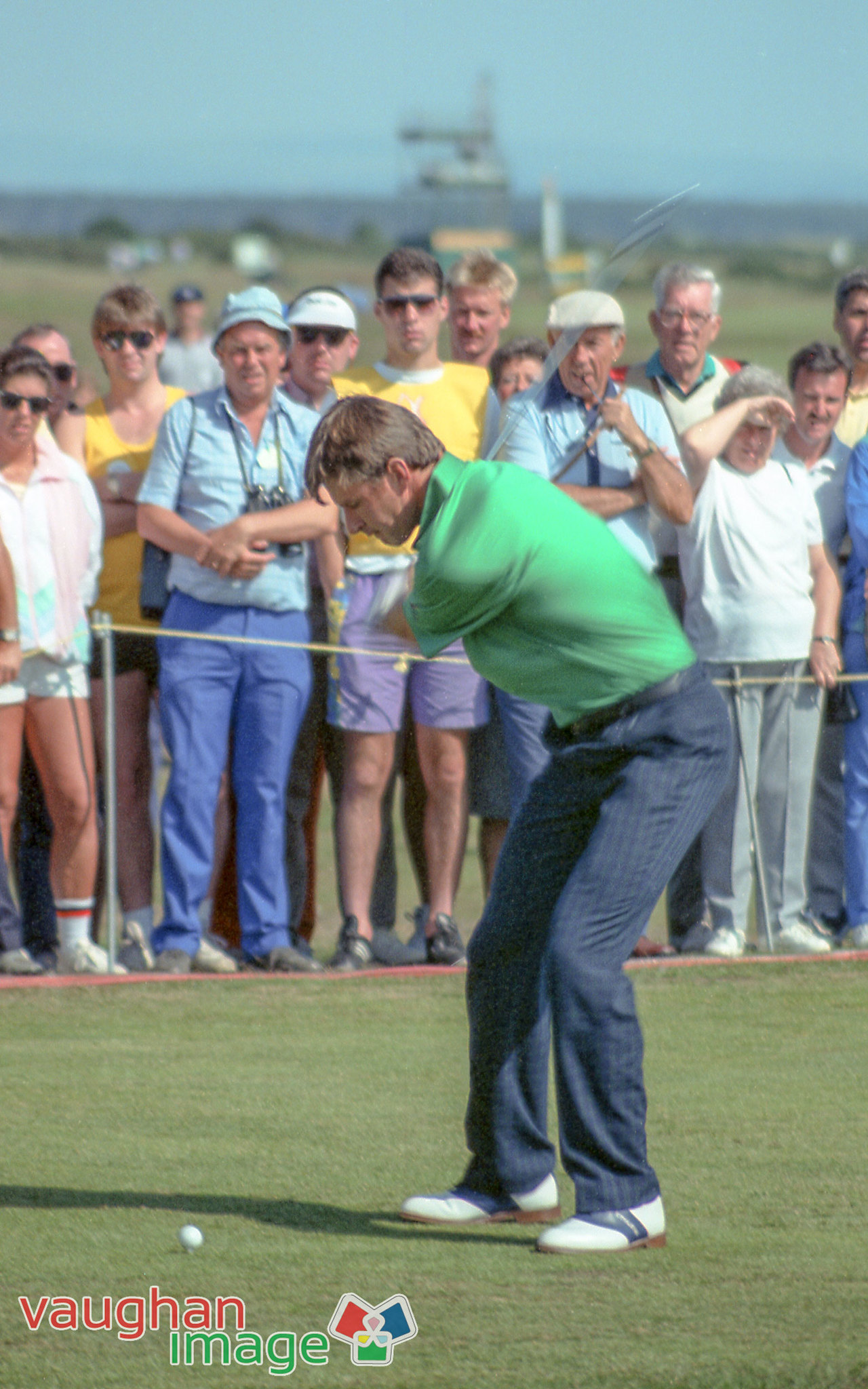The image captures a golfer mid-swing, raising his slightly blurred club, with a ball perched on a tee in front of him. He is wearing a vivid green shirt tucked into blue pinstriped pants, complemented by mostly white dress shoes with blue accents. In the background, a rope barrier separates him from a crowd of spectators, who are predominantly middle-aged and older, though a few younger individuals are also visible. Beyond the spectators, the sky and the surrounding landscape stretch out. In the bottom left-hand corner, a logo reading "Vaughan Image" is present, featuring three colorful cards: red pointing top left, blue pointing top right, and green pointing downward.